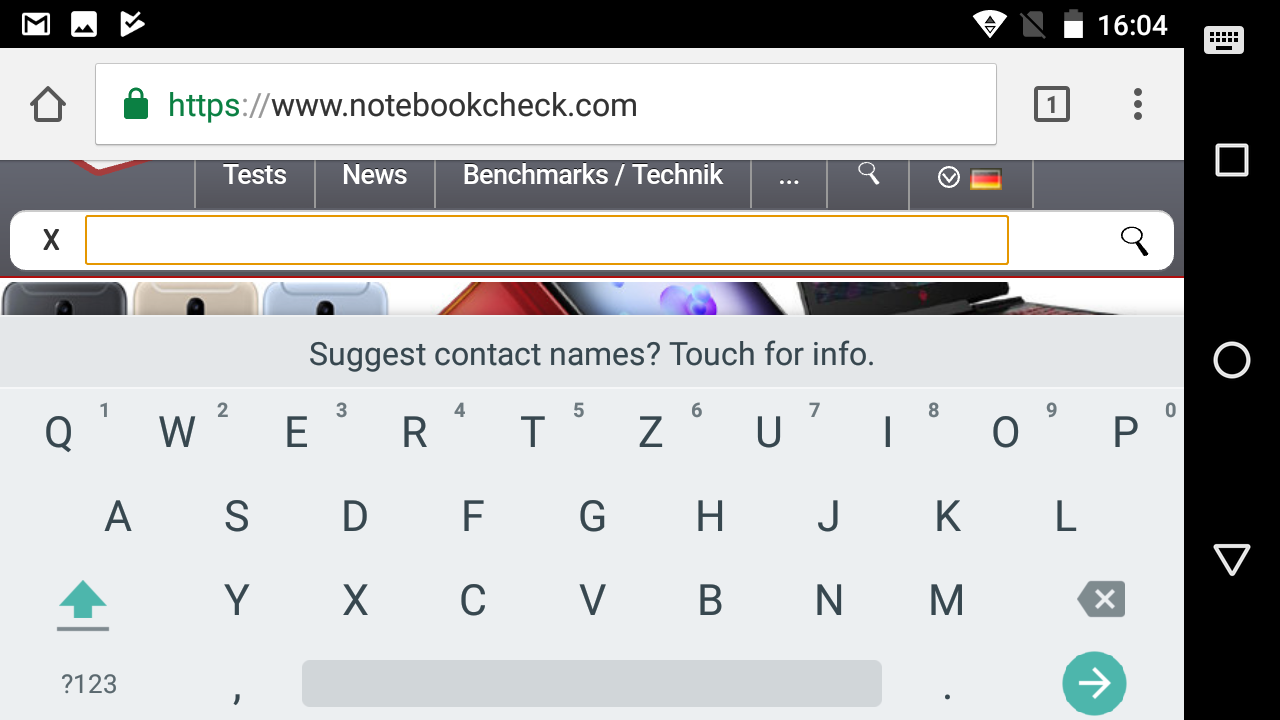The image is a screenshot of a website captured on a mobile device. At the top of the image, there's a thin black bar that also extends down the left side. At the upper left corner of this bar, white icons are visible: the Gmail icon, a mountain scene within a square (likely the Photos app), the Google Play Store icon, a Wi-Fi symbol, a battery symbol, and the time shown as 16:04.

Below this black bar, there is a visible thin gray navigation bar containing a black house icon, a white web address bar with a green padlock next to "notebookcheck.com," and a small window icon with a number "1" next to it, followed by three vertical gray dots.

Further down, a menu bar in varying shades of gray and white lists sections such as "Test," "News," and "Benchmarks/Technique." This menu also includes three dots, a magnifying glass icon, and a flag colored in black, red, and gold.

The next section features another search box with an orange outline, an 'X' for canceling the search, and another magnifying glass icon. Below this, the top portion of the main content area displays partial images of several electronic devices in different colors: black, gold, powder blue, and burgundy. The background includes a vibrant wallpaper in shades of purple and blue.

At the bottom of the screenshot, there is a white keyboard with gray keys, presented with the text "This keyboard suggests contact names, touch for info." The keyboard keys feature black text, and it includes notable elements such as a teal arrow, a gray spacebar, and a teal circle with a white arrow inside it.